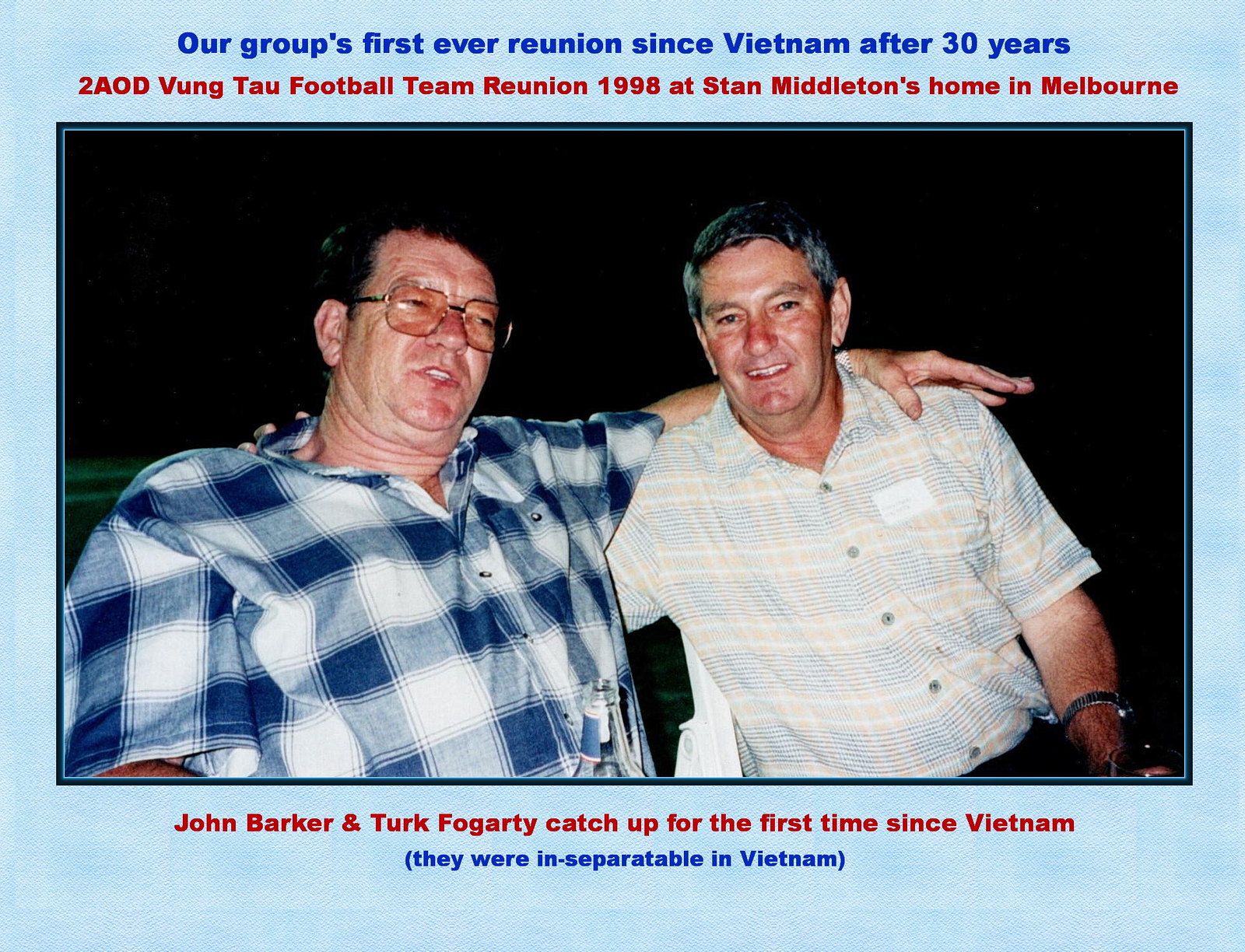The image captures two middle-aged men at their group's first reunion after 30 years since serving in Vietnam. This event, the 2AOD Vung Tau Football Team Reunion, took place in 1998 at Stan Middleton's home in Melbourne. The man on the left, a white individual with dark black hair, a pale face tinged with redness, and large glasses with a light pink tint, is wearing a blue and white checkered short-sleeved button-up shirt. He has his arm affectionately draped over the man on the right, who is also white, with grayish hair parted to the left, a slightly open mouth showing his teeth, and dressed in a creamy and beige short-sleeved shirt adorned with grey lines. This heartwarming photograph, set against a blue background, depicts John Barker and Turk Fogarty reuniting for the first time since their inseparable days in Vietnam. Additionally, a white card is visible on the right man's chest, and it appears he might be holding a bottle, possibly beer.